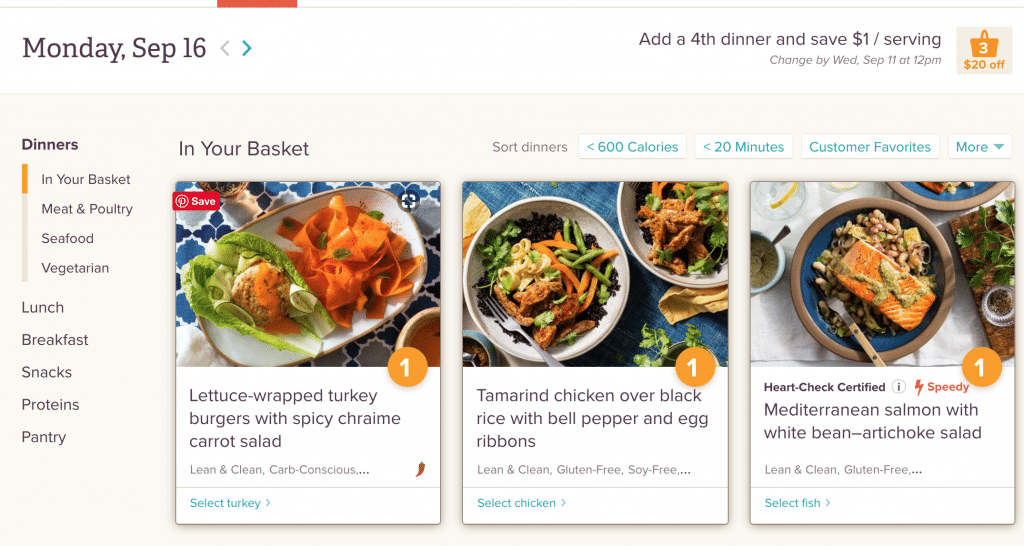This image is a screenshot of an online meal ordering system displayed on a computer screen. At the top left corner, the date "Monday, September 16th" is visible, accompanied by navigation buttons to move backward and forward. The back button is faint, indicating it is not active, while the forward button is highlighted in blue. There is an option that reads "Add a fourth dinner and save $1 per serving," with instructions to change the order by "Wednesday, September 11th at 12 p.m."

In the upper right corner, there is an orange basket icon with the number "3" in white, alongside the message "$20 off" in orange. The basket signifies that three items have been added.

Displayed under the label "In Your Basket," the selected dinners include:

1. Lettuce-Wrapped Turkey Burger with Spicy Crème Carrot Salad
2. Tamarind Chicken over Black Rice with Bell Pepper and Egg Ribbons
3. Mediterranean Salmon with White Bean Artichoke Salad

Each dinner listing has an orange circle with the number "1," signifying the quantity added to the basket. 

Further options available for selection are categorized under "Meat & Poultry," "Seafood," "Vegetarian," and additional categories such as "Lunch," "Breakfast," "Snacks," "Proteins," and "Pantry." These categories are meant for easy navigation and selection of meal types and items.